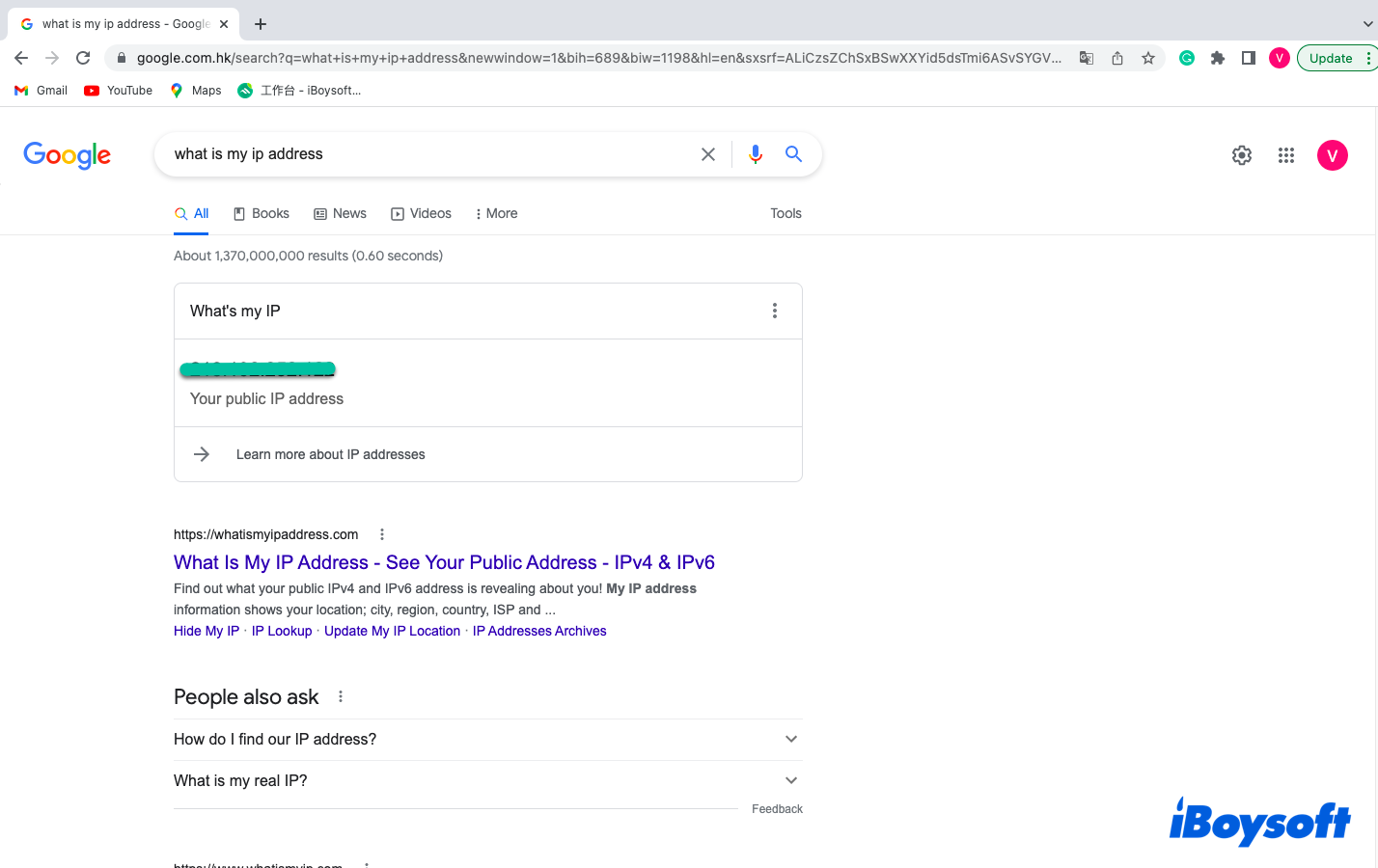The image depicts a computer screen with a white background, showcasing a browser window. At the top of the screen, there's a long gray rectangular bar containing a tab that displays a Google icon and the text "What is my IP address?". Below the tab bar, common browser navigation buttons are visible: a back arrow, forward arrow, and refresh button, followed by an address bar and various icons on the right-hand side including Gmail, YouTube, Maps, and another Google icon.

The search query "What is my IP address" is clearly typed in the search bar. Below the search bar, a horizontal navigation menu features options like All, Books, News, Videos, and More, with "All" being highlighted. The main content area displays the phrase "Your public IP address" in a seafoam green highlight, accompanied by a link labeled "Learn more about IP addresses" and another clickable blue link, "What is my IP address?".

Additionally, the section includes commonly asked questions such as "How do I find our IP address?" and "What is my real IP?". There is a feedback option on the right-hand side and a mention of "Boy Soft" in blue text towards the far right.

Overall, the image captures a detailed view of a computer screen displaying a browser window actively searching for information regarding a public IP address.